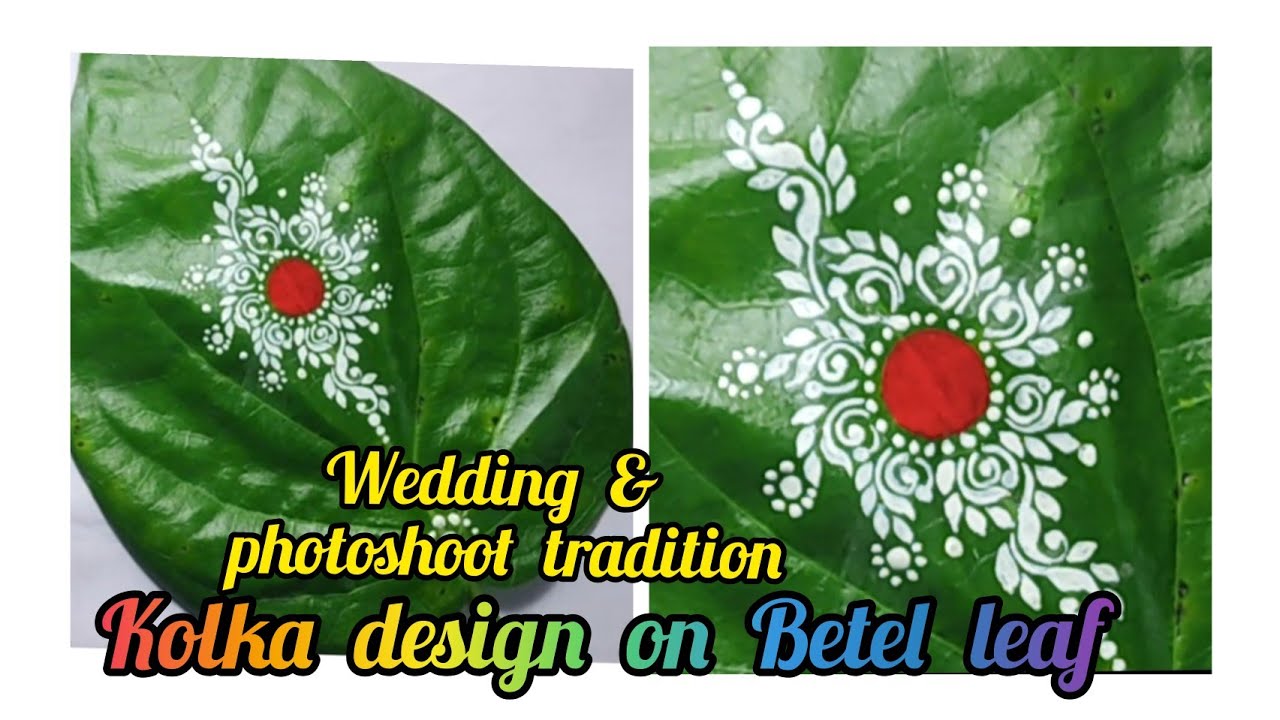The provided image is a diptych featuring a bright green betel leaf with a detailed coca design. The left side showcases the entire leaf, adorned with a red circular center encircled by ornate white floral patterns. The right side offers a close-up of the same intricate design, highlighting additional small white circles and extending floral motifs. A white bar separates the two images. Overlaying the left image, in yellow cursive lettering with a black outline, are the words "Wedding & Photoshoot Tradition." Along the bottom of both images, the text "Coca Design on Betel Leaf" is displayed in a gradient rainbow pattern transitioning from red to orange, yellow, green, blue, and purple. The images are well-lit, vivid, and clearly emphasize the traditional and decorative aspects of the coca design on the betel leaf.